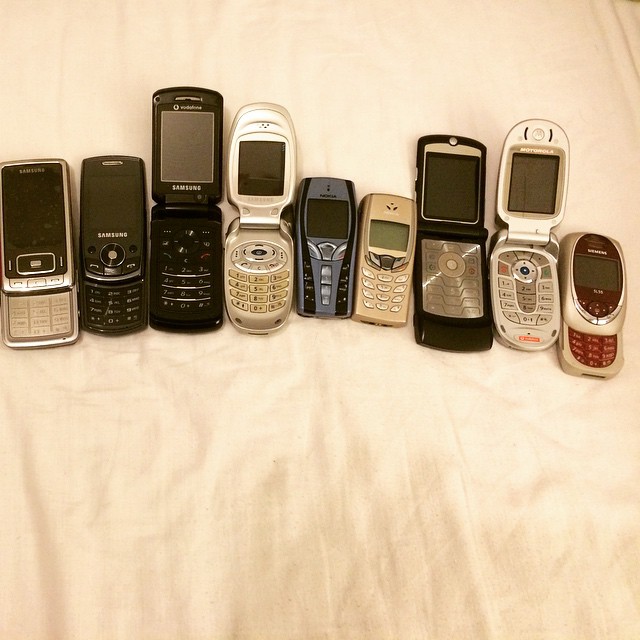The image showcases a collection of 11 vintage cell phones arranged in a single row on a slightly wrinkled off-white tablecloth, with the height of the image slightly exceeding its width. The phones consist of various types, including flip phones, slider phones, and classic brick-style phones, presenting a nostalgic array of monochrome screen devices.

From left to right:
1. A silver Samsung slider phone with a black screen.
2. A black Samsung slider phone.
3. A black Samsung flip phone.
4. A silver flip phone, potentially an LG model.
5. A blue and black Nokia brick-style phone.
6. A silver phone, likely another Nokia model.
7. A black and silver Motorola Razr flip phone.
8. A silver Motorola flip phone.
9. A silver slider phone with a red keypad, possibly a Nokia.

The arrangement and diversity in phone models and colors, including black, silver, blue, and red, create a visually interesting array set against the simple fabric background. The fabric displays vertical wrinkles, adding texture to the composition.